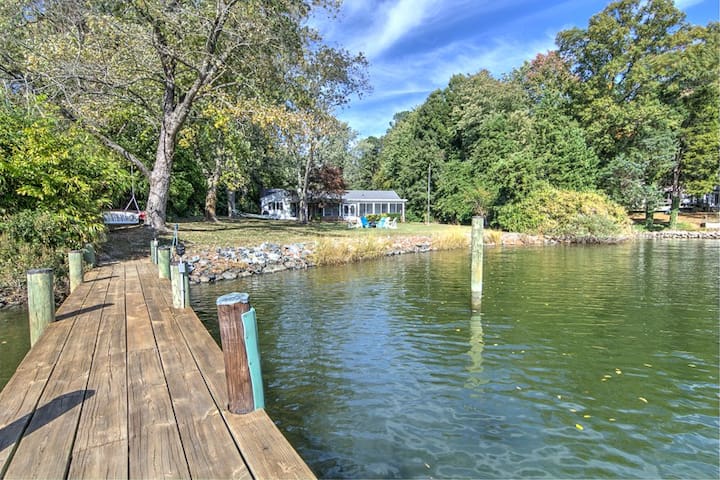The image captures a serene lakeside scene, characterized by a peaceful and rustic ambiance. To the left, a narrow, wooden pier extends into the distance, adorned with posts along its edges, inviting a tranquil stroll. The right side features a small, calm lake with a greenish hue, gently rippling and dotted with floating yellow leaves. This body of water is bordered by a rocky shoreline, lined with scattered stones. In the distance, a modest house with gray roofing and white or gray siding stands on the plot of land, contributing to the tranquil setting. Surrounding the house, an abundance of trees creates a dense, green backdrop, with some trees slightly yellowing, indicative of late summer. Among these trees, a hammock and a swing extending from their branches offer spots for relaxation. The sky above is a vivid, deep blue, accentuated by scattered, wispy white clouds, all bathed in bright, sunny daylight.